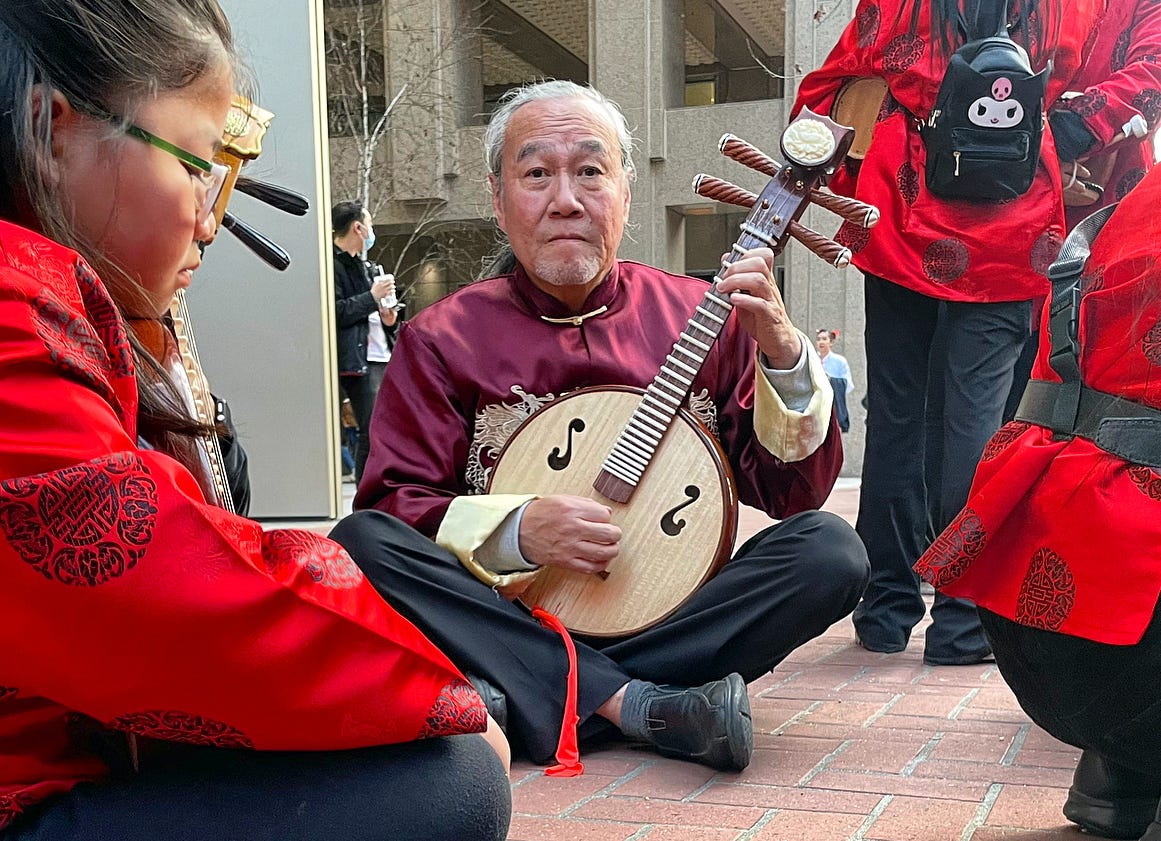In this vibrant, detailed color photograph, an elderly Asian man sits cross-legged on a brick-paved ground at the center of a bustling cityscape. He is dressed in a burgundy top featuring a mandarin collar, complemented by black pants and shoes. The man is deeply engaged in playing a unique stringed instrument that resembles a wooden banjo with several items protruding from its head. 

To his right, several people, presumably fellow musicians, are visible from the back, donning black pants and red blouses adorned with a Chinese motif. One of them carries a black backpack. Also on his right, a woman sits in profile to the camera, wearing a similar red blouse and glasses. She appears to be playing a similar stringed instrument, although it is mostly obscured from view.

In the background, a cityscape unfolds with large buildings looming and people meandering on the sidewalk. Among the pedestrians, one person dons a Kawaii-style backpack and a face mask, highlighting the lively and modern urban environment. The scene captures a harmonious blend of traditional musical artistry and the dynamic, contemporary city life.